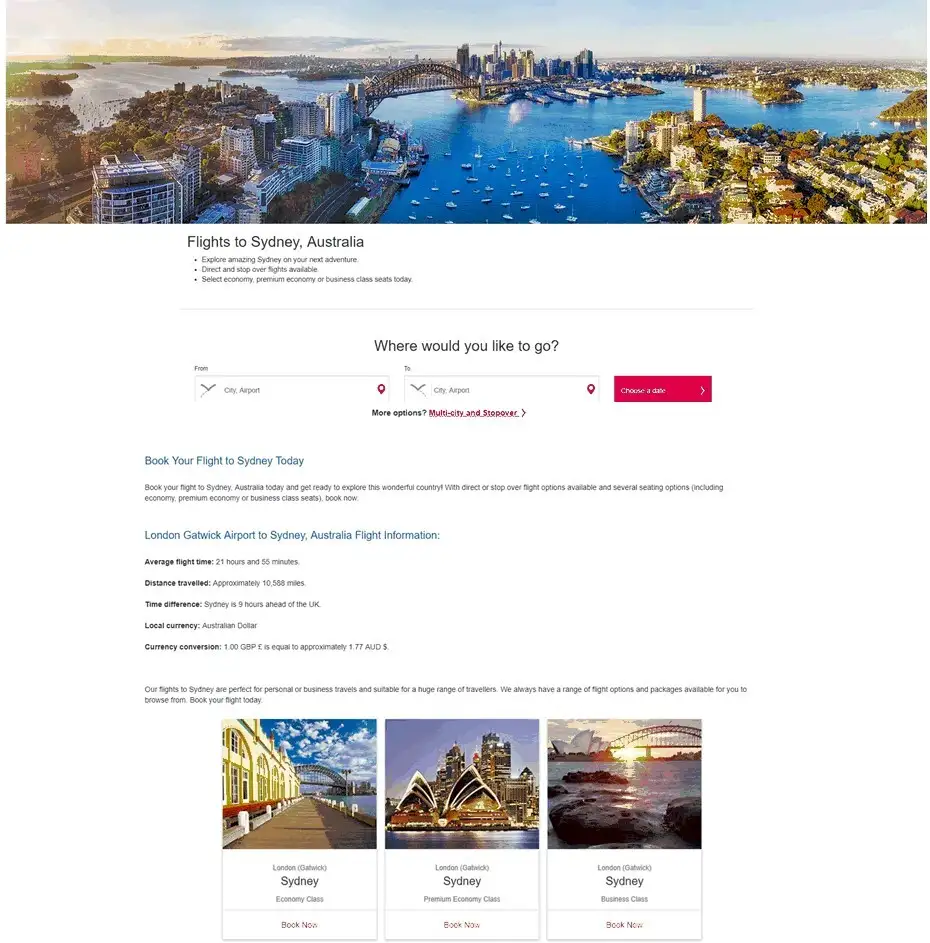This is a detailed flight booking page for trips to Sydney, Australia. The top of the page features a stunning panoramic image of Sydney. The aerial view captures the vibrant Sydney Harbor with its iconic curved bridge, bustling with boats. The view highlights the city's contrast of towering skyscrapers on the left and charming residential buildings on the right under a clear blue sky.

Below the image, the text reads "Flights to Sydney, Australia" in bold black letters, followed by an enticing call to action: "Explore amazing Sydney on your next adventure. Direct and stopover flights available. Select economy, premium economy, or business class seats today."

Further down, there's a question prompt, "Where would you like to go?" accompanied by two search boxes for departure and destination airports. A striking red button labeled "Choose a date" invites users to select their travel dates. Additional options such as "More options", "Multi-city", and "Stopover" are presented with a directional arrow for extended navigation.

The page also reinforces the booking message with a blue text line: "Book your flight to Sydney today." Black text underneath summarizes on how to proceed: "Book your flight to Sydney, Australia today, and get ready to explore this wonderful country with direct or stopover flight options available and several seating options, including economy, premium economy, or business class seats. Book now."

Detailed information about flights from London Gatwick Airport to Sydney, Australia is also provided:
- Average flight time: 21 hours and 55 minutes.
- Distance traveled: approximately 10,588 miles.
- Time difference: Sydney is nine hours ahead of the UK.
- Local currency: Australian dollar.
- Currency conversion: 1 Great Britain pound = approximately 1.77 Australian dollars.

The page concludes with three enticing images showcasing various attractions in Sydney, encouraging travelers to envision their journey.